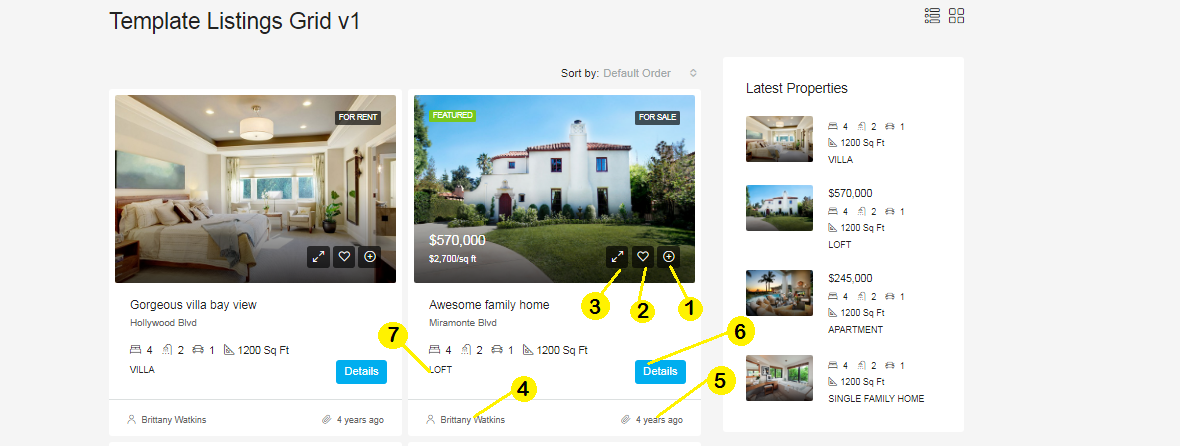Displayed on the website are images of various rental and for-sale properties. The image on the left features a spacious bedroom with a large bed adorned with numerous pillows and a beige comforter. Above the bed hangs an elegant painting, and a sizeable window offers a pleasant view. To the right, there's a listing for a sizable, two-story white home priced at $570,000, described as an "awesome family home" and complemented by a well-kept yard. Further to the right, labeled as "Latest Properties," are more listings: a 1,200 square foot villa, a 1,200 square foot apartment, and a single-family home notable for its numerous windows.